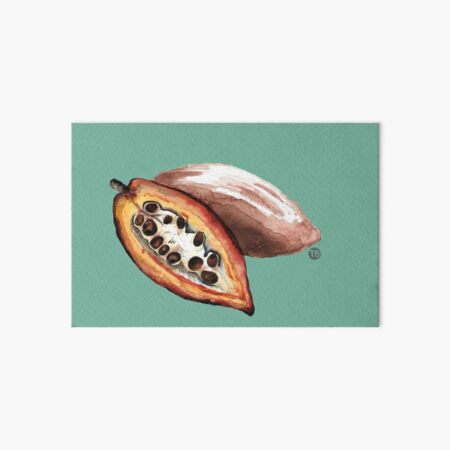The image is a painting displayed on a solid white wall, depicting two papayas against a teal or sea green background. The focal point is a sliced-open papaya positioned in the front, revealing its intricate insides. The fruit's red outer flesh transitions to a yellow inner layer, encasing a core filled with rows of large brown seeds set in a white area. The cut papaya also features a visible stem. Behind it, a whole, elongated papaya with a brownish-tan skin leans into the scene. A watermark, consisting of the letters "TB" inside a brown or black circle, is situated near the bottom right corner of the painting. The composition highlights the detailed and naturalistic portrayal of the fruit, accentuating the muted yet rich colors.